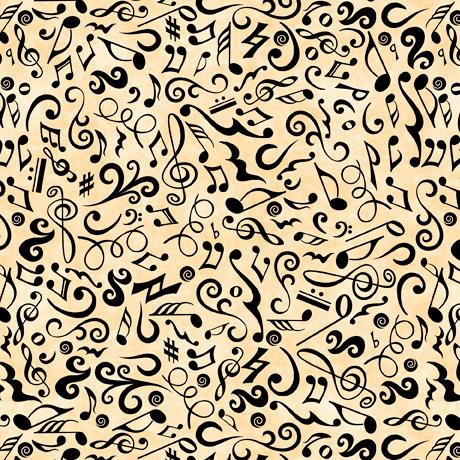This image features a decorative art piece on a taupe, tan-ish, cream-ish textured background, densely covered with an array of black musical notes and symbols. The musical elements vary in sizes and directions, creating a dynamic and somewhat chaotic arrangement. Among the assortment, you can identify large treble clefs, small notes, rests, crescendos, and even hashtag-like symbols. Some of these notes and symbols stretch beyond the borders of the image, giving it an incomplete and abstract feel. The overall composition, with its mix of swirls, squiggles, and various musical notations, evokes a design that would be well-suited for decorative purposes such as on fabric or wallpaper.